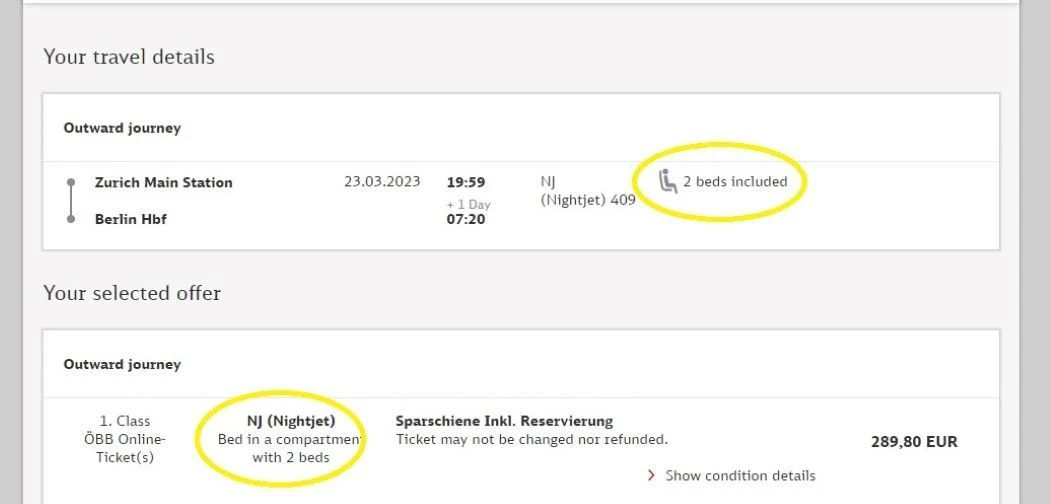Screenshot of Travel Itinerary: 

A detailed screenshot taken from a computer, showcasing travel tickets for a journey. The interface has a rectangular shape, indicating it's likely captured from a laptop or desktop. The background of the screenshot is light gray with black text. 

At the top, the text reads: "Your Travel Details". Below, two white boxes contain specific information about the journey. 

In the first white box, under "Outward Journey", the details provided are:
- Departure: Zurich Main Station
- Destination: Berlin HBF
- Date: 23-03-2023
- Departure Time: 19:59
- Arrival Time: 07:20 (next day, +1 day indicated)
- Service: NJ (Night Jet) 409
- Included Amenities: two beds

The journey appears to be a night train service, as noted by the inclusion of two beds, suggesting a comfortable overnight trip. The selected offer details are also mentioned: "Outward Journey, 1st Class, OBB Online Ticket, NJ (Night Jet), Bed in compartment with two beds."